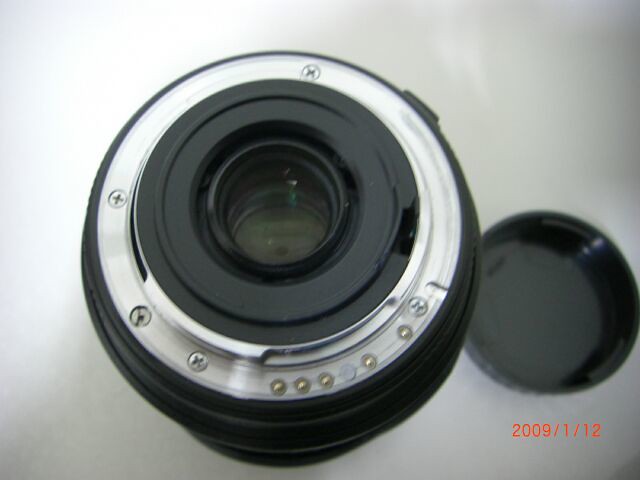This is a color photograph centered on a dismounted camera lens, predominantly featuring black, silver, and gray hues. The lens, positioned on a white surface with slight shadows around its edges, offers a nearly head-on view with a slight tilt revealing some depth. The core of the lens showcases a glass element encircled by a black plastic ring. Surrounding this is a circular silver metal rim adorned with several Phillips head screws. Further out, another ring of black plastic completes the primary structure of the lens. To the right of the lens lies a black plastic lens cap, overturned. In the bottom right corner of the image, an orange timestamp reads "2009-1-12," marking the date of the photograph.